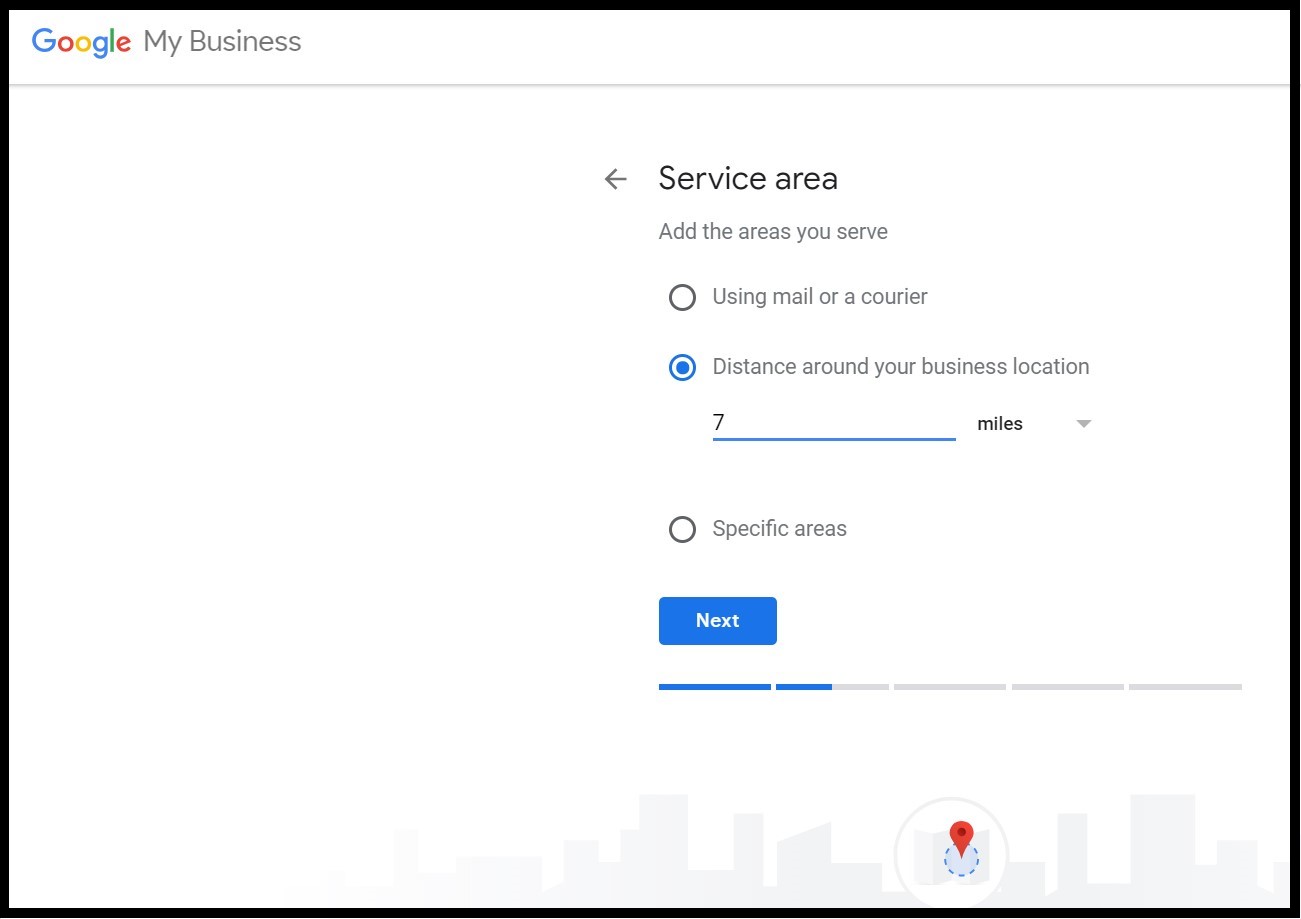This is a screenshot of a Google My Business setup page. The iconic Google logo is displayed at the top, featuring its traditional blue, red, yellow, blue, green, and red colors. Directly beside it is the "My Business" text in gray. Below this header, there's a gray back arrow indicating navigation options.

The current section is labeled "Service Area," prompting users to "add the areas you serve." The background throughout the page is white, providing a clean and clear interface. Users are presented with three options to define their service area: 

1. "Using mail or a courier"
2. "Distance around your business location"
3. "Specific areas"

At present, the "Distance around your business location" option is selected, with a typed input of "7 miles." There is also a drop-down menu, likely allowing the choice between miles and kilometers, although this is not confirmed.

Beneath this section lies a progress bar with five segments, indicating that the user has completed the first step and is currently on the second step of the setup process. 

At the bottom of the screenshot, a light gray outline resembling a cityscape is visible, along with a red pinpoint icon whose exact function or location is unclear.